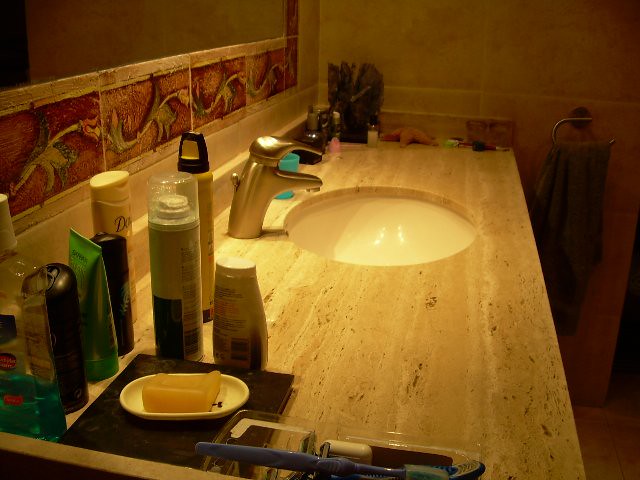The image depicts a well-organized bathroom sink cabinet area. The counter itself is a sleek straight-edged design, possibly made from a wooden or marble material. Centrally placed is a circular, sunken sink with a modern faucet featuring a single lever that controls both hot and cold water. 

The countertop is adorned with various bathroom essentials: a can of mousse, a container of shaving cream, a bottle of Dove body wash, mouthwash, soap, a toothbrush, dental floss, deodorant, and assorted lotions and creams. There is also a whimsical assortment of decorative items including a starfish, a small plant, additional small tubes and bottles, a blue cup with a pink lid, giving the counter a personalized touch.

Above the sink hangs a mirror framed by rustic, reddish floral tiles, enhancing the aesthetic appeal of the space. A towel bar attached nearby holds a beige-brown towel, adding warmth to the setting. The walls are tiled with large, greyish-cream tiles, contributing to a clean and contemporary look. Overall, the bathroom exudes a cozy yet stylish ambiance with its mix of essential items and decorative touches.